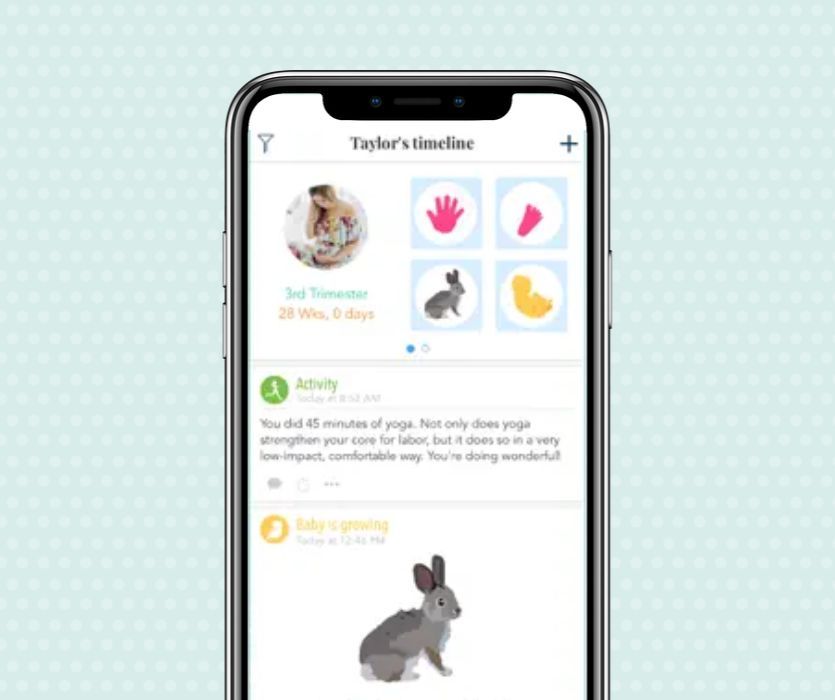A slightly blurry photograph captures a smartphone displaying a screenshot of a user interface, set against a light mint green background with a subtle circular hatched pattern. The smartphone, which takes up approximately three-quarters of the image, has a dark gray edge. Visible in this shot are two side buttons on the left, a single button on the right, and a camera module at the top featuring two lenses flanked by a speaker.

The app displayed on the phone has a white background header labeled "Taylor's Timeline." On the left side of the header, a pin-like or menu icon is visible, while a plus symbol appears on the right. Below this header is a gray line break followed by a circular profile picture of a light brown or dirty blonde-haired woman, who appears to be pregnant and Caucasian, though the low resolution obscures finer details.

Adjacent to the profile picture, there are four icons arranged in two rows of two: a hot pink hand and foot on the top row, and a gray bunny alongside what looks like a yellow fetus icon on the bottom row. Below the profile picture, green text indicates "Third Trimester," followed by "28 WKS, 0 days" in orange. Two navigation tabs are below this, one blue and filled to indicate it's selected, the other outlined in blue but unfilled.

Further down, a green card displays an icon of a person running, labeled "Activity," with a timestamp and message stating, "You did 45 minutes of yoga. Not only does yoga strengthen your core for labor, but it does so in a very low-impact, comfortable way. You're doing wonderful." 

At the bottom, another section showcases a yellow fetus icon next to text that reads "Baby's Growing," with a timestamp showing today at possibly 12:42 p.m., though it's difficult to be certain. Finally, a gray rabbit graphic indicates the size of the baby at this stage of gestation. Icons for comments, sharing, and a three-dot menu hint at additional interactions, although they are hard to discern clearly due to the image's low resolution.